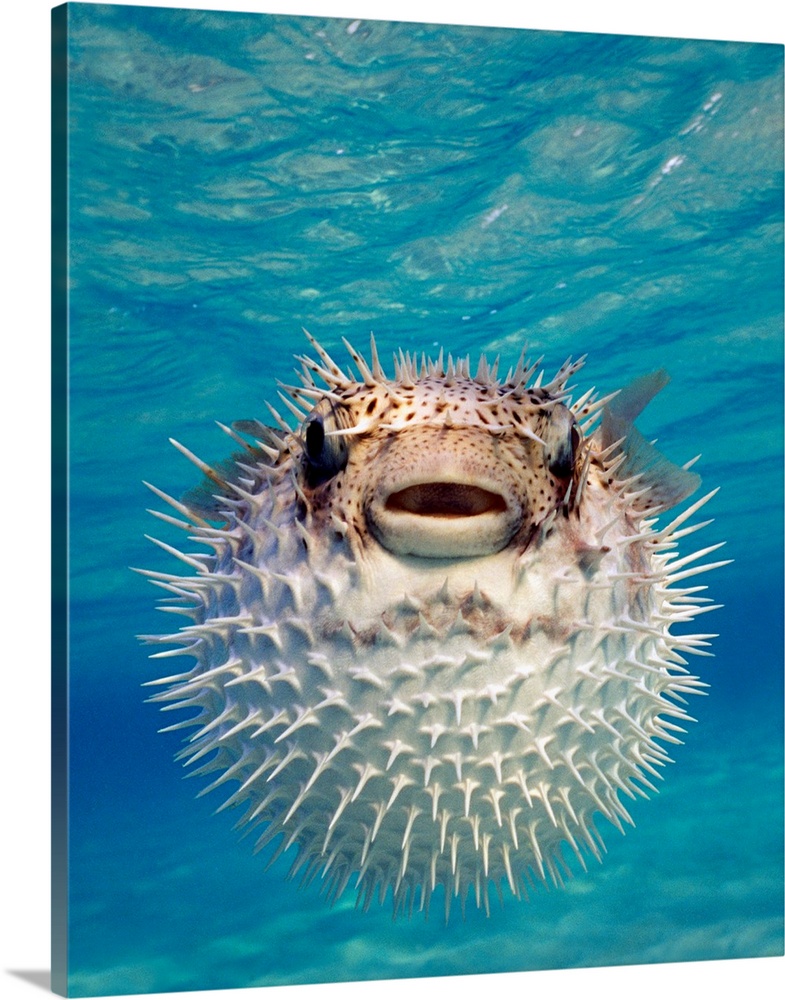This image, a detailed photograph printed on a canvas, displays a central, fully puffed-out puffer fish, framed in a square rectangle setup, reminiscent of photo canvases seen at retail photo centers. Facing directly towards the camera, the puffer fish appears dominant in the clear, blue ocean. Its body is speckled with brown spots, with white trim and black eyes, while its spiked portions are also white. The fish's mouth is open, and its eyes are wide, giving a vivid sense of alertness. The underwater scene reveals a sandy ocean floor with no other sea creatures visible, emphasizing the puffer fish as the sole subject. Above, the water surface is slightly rippled, capturing the essence of a clear ocean environment. The canvas itself is slightly tilted forward to the left, casting a subtle shadow behind it, but there is no text associated with this pristine aquatic portrayal.